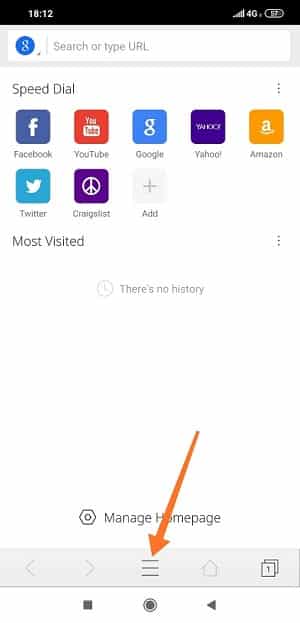The image is a screenshot taken from a smartphone. At the top of the screen, there is a Google emblem and a search bar. Below the search bar, the screen features a "Speed Dial" section, which displays several shortcut icons to popular websites. These shortcuts include Facebook, YouTube, Google, Yahoo, Amazon, Twitter, and Craigslist. Each of these icons has distinct colors: Facebook in dark blue, YouTube in red, Google in blue, Yahoo in purple, Amazon in a yellowish color, Twitter in light blue, and Craigslist in its usual format.

The section titled "Most Visited" appears in gray text below these icons. There is also a small clock icon labeled "History" nearby. Dominating the center of the screen, a large orange arrow points diagonally downward towards a group of vertical lines. Beside these lines, the text reads "Manage Home Page." Below this, there is a "Copy" button. At the very bottom of the screenshot, there are three navigation icons: a triangle, a circle, and a square. The overall layout is designed to provide quick access through visual and textual cues.